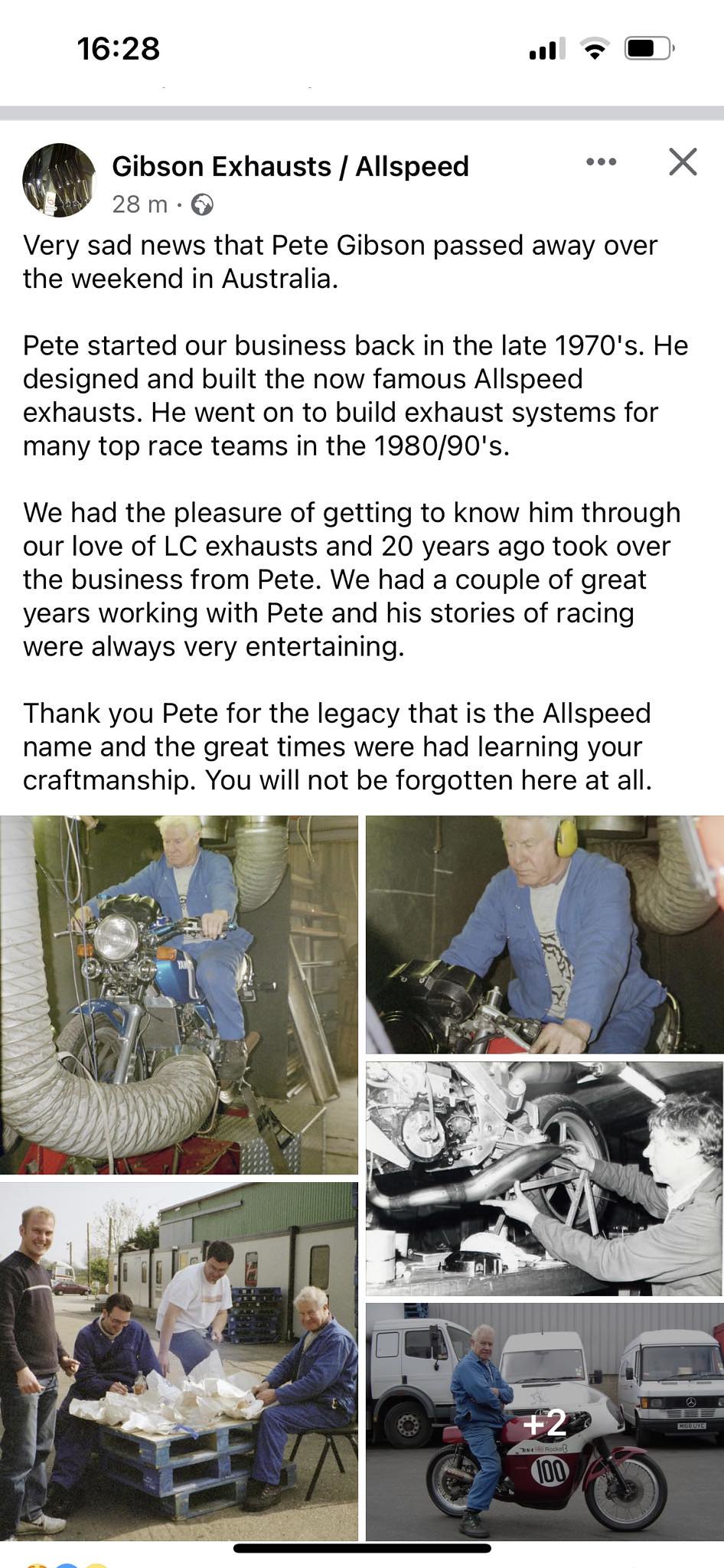This detailed, full-color screenshot appears to be a memorial post from a social media platform, possibly Facebook or Twitter, dedicated to Pete Gibson. The image prominently displays phone information at the top, including a timestamp of 16:28, three of four bars for wireless connectivity, two of three bars for Wi-Fi connectivity, and a half-full battery icon. Below this, a grey line separates the phone details from the actual content. The post is from "Gibson Exhaust / All Speed," created 28 minutes ago, and marked with a globe icon indicating public visibility.

The post expresses very sad news that Pete Gibson passed away over the weekend in Australia. Pete was the founder of Gibson Exhausts and started the business in the late 1970s. He was well-known for designing and building the famous All Speed Exhaust systems and contributed significantly by crafting exhaust systems for top race teams during the 1980s and '90s. The company mentions taking over the business from Pete 20 years ago and reminisces fondly about the great times and entertaining racing stories Pete shared. His legacy in craftsmanship and the All Speed name remains cherished and unforgettable.

At the bottom of the post, there are several photographs of Pete Gibson at different stages of his life. The first image shows him in a blue coverall, with gray hair, riding a motorcycle in a shop; the motorcycle is fitted with a large exhaust tube. Another close-up image features Pete with yellow hearing protectors. There's also a black and white photo of Pete working on an exhaust manifold, exemplifying his hands-on craftsmanship. Additional photos capture him enjoying moments with colleagues; one shows him sitting around makeshift tables with three other men, and another depicts him on a red motorcycle numbered 100, with an overlay suggesting more photos can be accessed by clicking. This post serves as a tribute to Pete Gibson's life and contributions to the motorcycle industry.